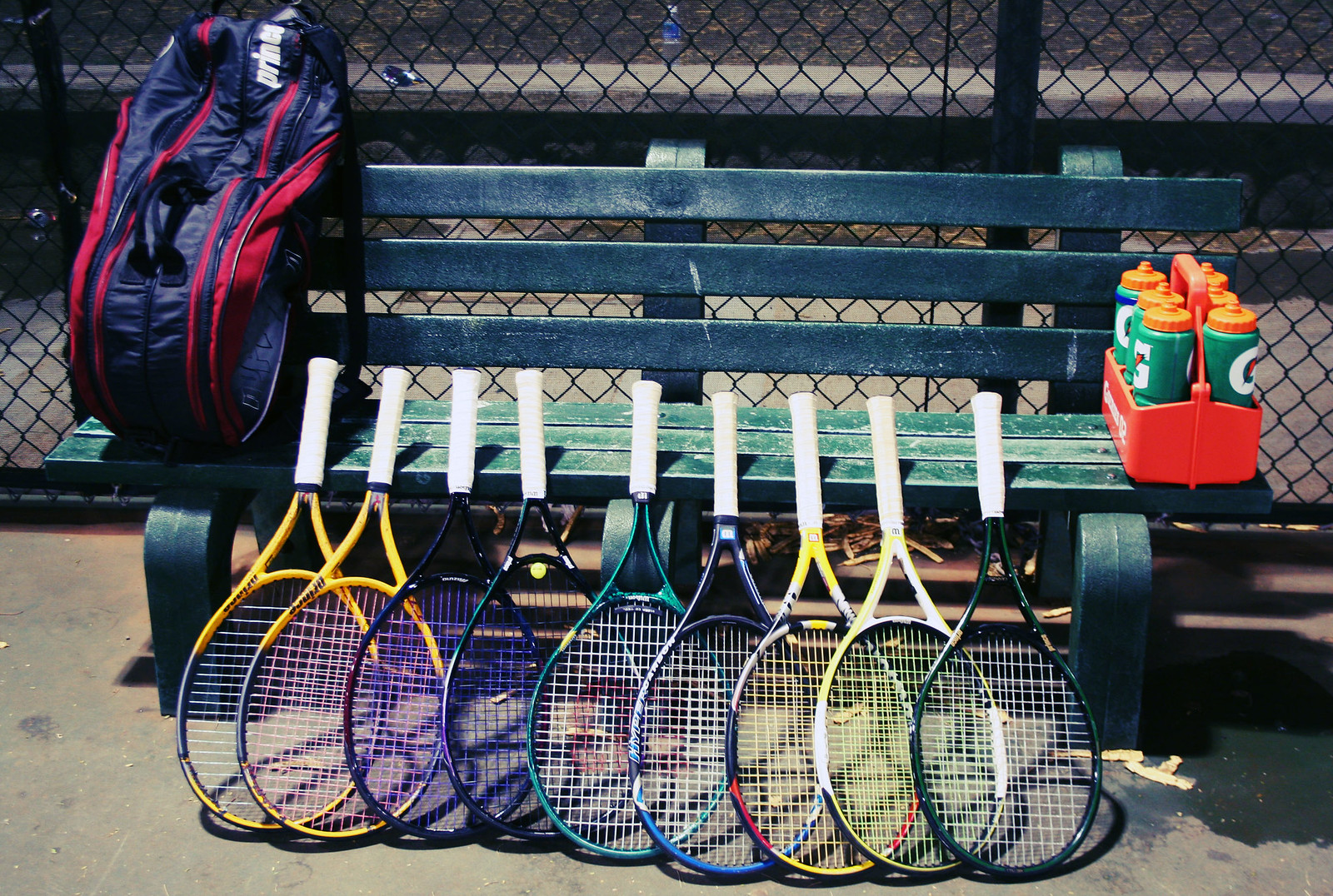This detailed photograph captures a well-arranged scene of tennis equipment at a park's tennis court. In the foreground, nine tennis rackets with white grips rest against a green slatted wooden bench supported by cement stanchions. The rackets, fanning out from left to right, display a variety of colors: yellow, black, green, blue, and multicolored, with the racket heads positioned on the ground. On the bench's left side, a navy blue and red tennis bag sits upright, while on the right, an orange Gatorade caddy holds six green bottles with orange caps, each marked with the iconic "G" for Gatorade. In the background, a black mesh fence encloses the area, and beyond that, a sidewalk is visible. Scattered around, an abandoned set of keys and a water bottle add a touch of realism to the meticulously composed shot, enhancing the impression of a candid moment frozen in time. The tall black fence surrounding the court emphasizes the setting's recreational and somewhat secluded environment.